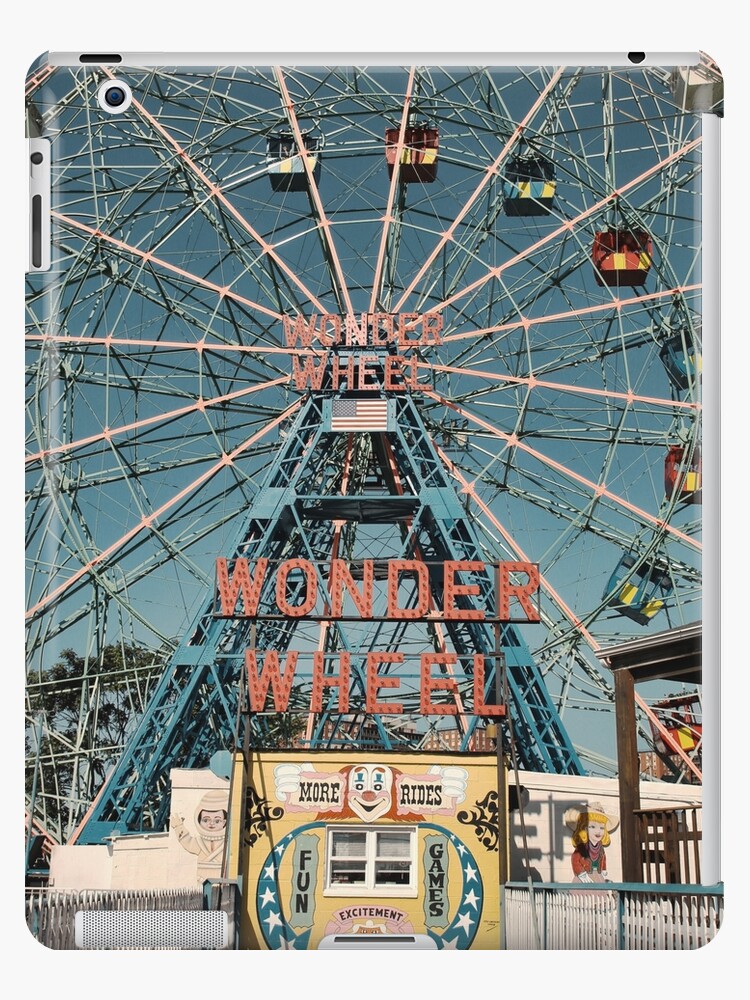The image showcases a towering Ferris wheel named "Wonder Wheel," dominating the frame with its grand presence. At its center, the "Wonder Wheel" signage is prominently displayed in red, with an American flag fluttering beneath it. The Ferris wheel is constructed of metal and features alternating carriages with green and yellow stripes in some and red and yellow stripes in others. Surrounding the Ferris wheel is a bustling carnival setting, complete with a ticket booth adorned with a clown face at the entrance. The booth has a white window and bears a sign reading "More Rides, Fun Games, Excitement." Fencing encircles the ride, enhancing the carnival atmosphere. Captured in broad daylight, the image also reveals glimpses of the carnival's vibrant details, including a trailer with a cowgirl logo on the right side. The background includes a light gray border, and its overall appearance is reminiscent of a vintage photograph, complete with beveled edges.